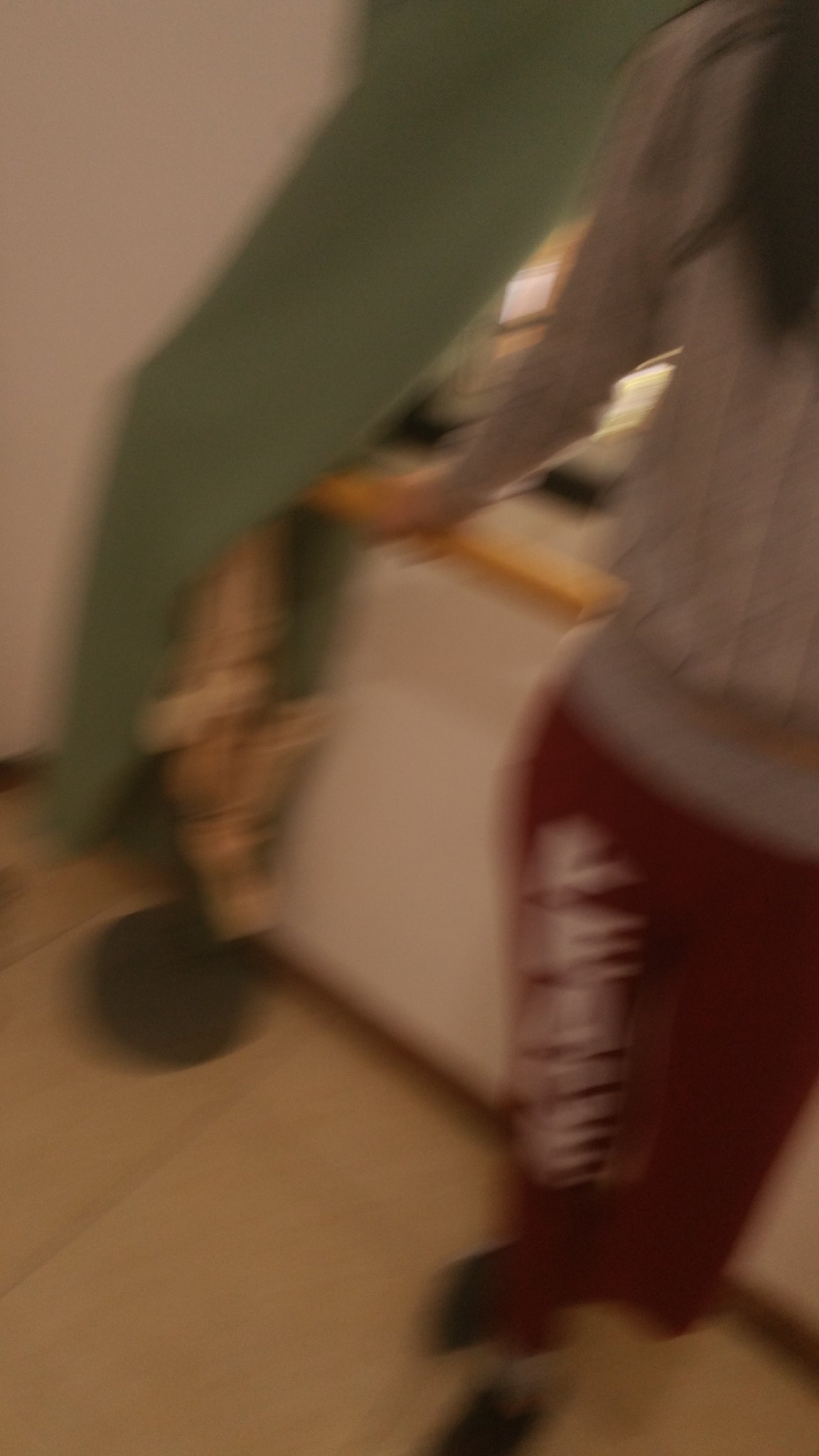A woman stands at a counter, potentially in a store or a bank, engaging in a customer service interaction. She wears beige pants and a long green shawl, leaning forward to speak with a representative. In the foreground, another woman, dressed in red sweatpants with white lettering on the left leg, and a gray sweater, is more prominently featured. She pairs her outfit with black shoes. The setting includes a rectangular-tiled floor and a gray wall, giving the environment a modern, utilitarian feel.